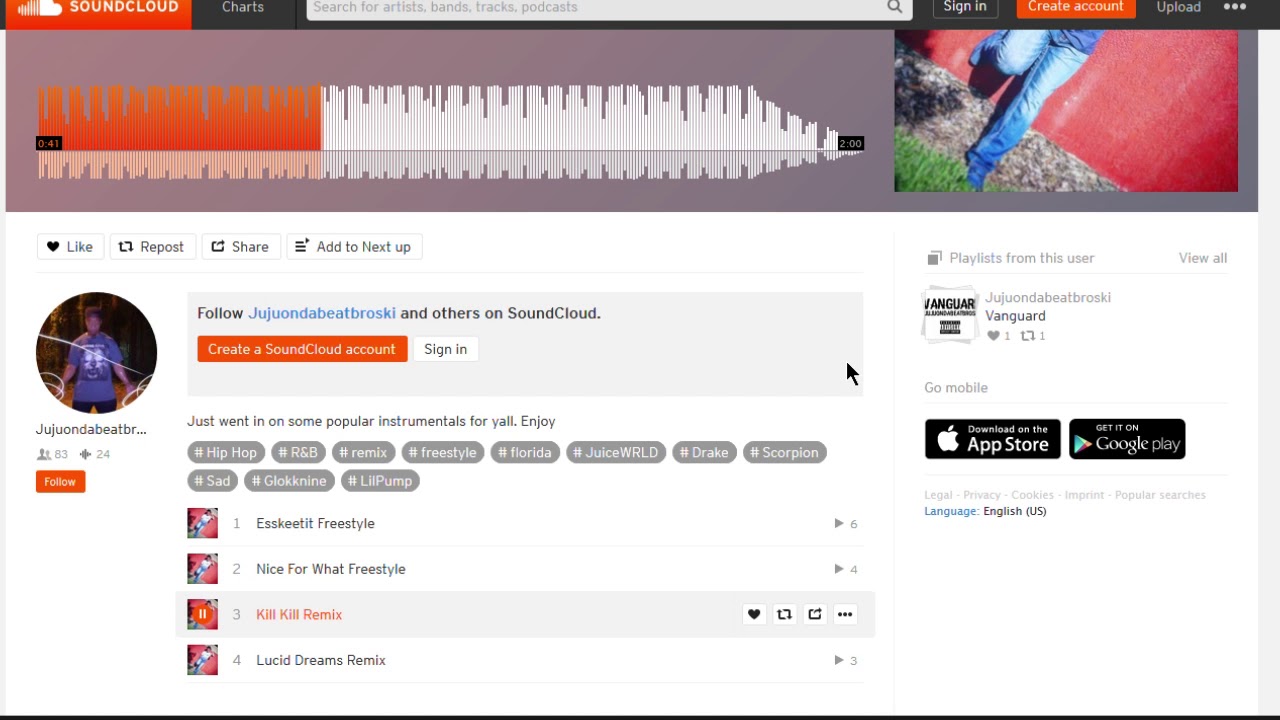**Screenshot Description: SoundCloud User Interface**

The screenshot depicts the SoundCloud user interface against a white background. Central to the image is a chart characterized by bar graphs that represent the volume levels of a song. The duration of the song is visible and is marked at two minutes and five seconds. The initial 41 seconds of the chart are highlighted in orange, distinct from the rest of the white chart.

The interface displays several standard SoundCloud elements:
- **Search Bar:** Located at the top, designed for finding tracks.
- **Sign In and Create an Account Options:** Prominently positioned for user access.
- **Upload Button:** Available for contributing content.
- **Three Horizontal Dots:** Indicating additional options.
- **Repost, Share, Add to Next Up, Follow, and a Hamburger Icon:** Functionalities for interaction with the track and user actions.
- **Profile Section:** Featuring a user's name, SoundCloud identification, and a prompt to create a SoundCloud account.
- **Popular Tags:** Including terms like "hip hop," "R&B remix," "freestyle," "Florida," "Juice WRLD," "Drake," "Scorpion," and "sad."

In the screenshot, an orange SoundCloud logo is noticeable, and descriptions like "create a SoundCloud account" and "sign in" are clearly displayed. The image also mentions popular instruments and trending tags, prominent in a visually clean white and orange thematic layout.

This comprehensive snapshot effectively captures the navigation and functionalities available to users on the SoundCloud platform.